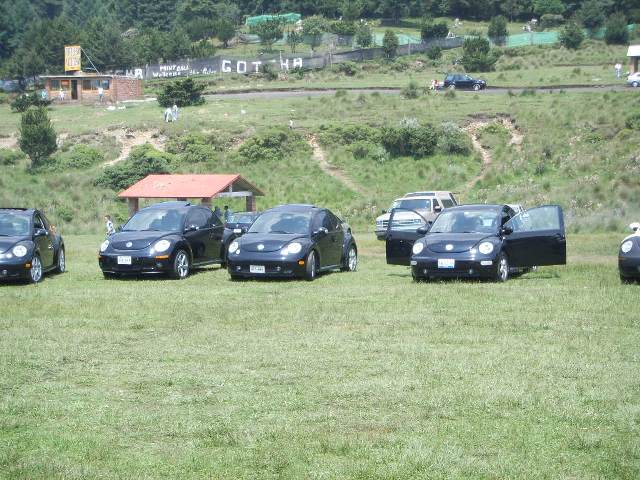In this outdoor photo, five black Volkswagen Beetles are arranged on a grassy field, all facing the camera slightly to the left. The fourth Beetle from the right has both of its front doors open. A couple of individuals, likely two adults, are positioned behind the second Beetle on the right, while children are visible near the second Beetle on the left. The background reveals a small hill leading up to a brown building on the left, which features an unreadable yellow sign. Behind the building and towards the right is an unmaintained dark brown dirt road, with a black vehicle further down and a silver sedan at the rightmost part of the road. Adjacent to the road is a net fence or gate displaying the word "GOTHA." Beyond these elements, there are green net gates and a dense, dark green forest. The image appears to be taken on a sunny day, but is somewhat grainy.